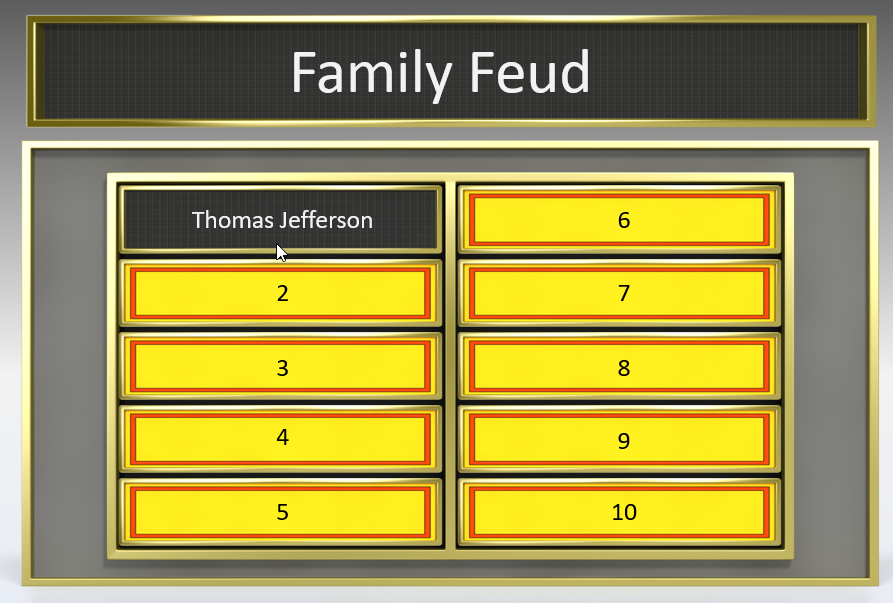The image depicts a scoreboard from a Family Feud game, likely from a computer or video game version. A large gray title bar at the top of the screen proudly displays "Family Feud" in white letters, framed by a shiny gold border that gives it an eye-catching look. Below the title bar, a gray rectangular area serves as the background for the answer board. This board is divided into ten vertical slots, arranged in two columns of five. Each of the slots, numbered 1 through 10, features a yellow background with a red outline. The very first slot, which stands out with its black background, prominently displays the name "Thomas Jefferson" in white text. Additionally, a white mouse cursor is seen hovering near the slot containing "Thomas Jefferson." The remaining nine slots are currently only numbered and not yet opened, awaiting further gameplay.